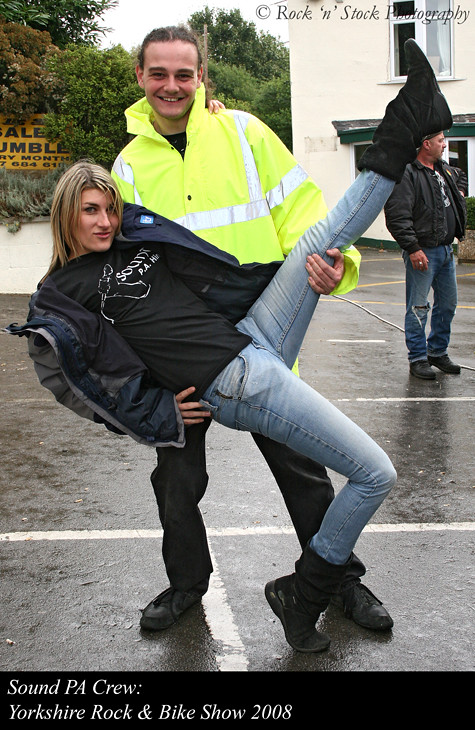The image captures an outdoor scene, likely shortly after or during rainfall, as the wet pavement suggests. Prominently featured are two people in a playful pose. A smiling man with long brunette hair stands at the back, wearing a lime green high-visibility jacket with reflective stripes, black trousers, and black shoes. He is supporting a woman who is leaning backwards into him, her left leg lifted into the air and held securely by the man's hand just under her knee. She balances on her right leg and has her arm wrapped around his shoulder. The woman, who has a mix of blonde and dark brown hair, wears a black t-shirt, light blue jeans, black boots, and a spring jacket that is open. Both are joyfully looking at the camera. In the background, a building with white-framed windows and a green entrance is partially visible, along with some trees and vegetation. To the right, another man dressed in jeans, a black jacket, and black boots is looking off to the side. The bottom of the image features a black banner with text that reads, "Sound PA Crew, Yorkshire Rock and Bike Show 2008," and the top right corner includes a watermark stating, "Rock in Stock Photography."